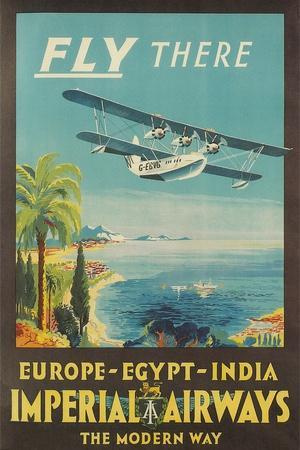This vintage travel poster, reminiscent of the prolific 1950s style, vividly captures the allure of tropical destinations. Against a clear blue sky, a classic white bi-winged airplane with three propellers flies over a pristine beach and turquoise lagoon. The airplane, marked with the small black letters "G-EGWG," carries the promise of adventure, as suggested by the bold white text "Fly There" at the top of the poster. Nestled in a picturesque tropical paradise, the scene below features lush palm trees, serene white-sanded shores, and distant boats dotting the tranquil waters. Majestic white mountains frame the horizon, enhancing the wild, untouched beauty of the setting. At the bottom of the poster, yellow lettering enthusiastically promotes the destinations served by Imperial Airways with the phrase: "Europe - Egypt - India. Imperial Airways: The Modern Way." The background is richly bordered in brown, adding a touch of nostalgic elegance to this enticing travel advertisement.